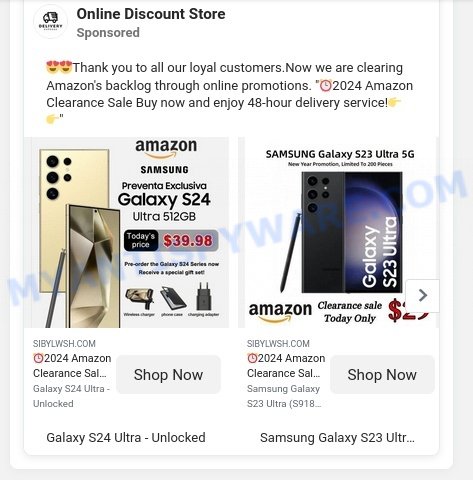**Sponsored Ad: Amazon 2024 Clearance Sale**

At the top of the ad, there's a prominent delivery truck icon featuring the word "delivery" as part of the logo. Below it, in grey text, it reads "sponsored." 

Centered on the ad are two smiley faces with heart eyes and the phrase: "Thank you to our loyal customers. Now we're clearing Amazon's backlog through online promotions."

A clock icon signals the "2024 Amazon Clearance Sale," with an urgent call to action: "Buy now and enjoy a 48-hour delivery service!"

To the right of this, there are several right-facing pointer hands drawing attention to two vertical ads below. 

**Ad 1:**
- Features the Amazon and Samsung logos.
- Promotes the "Preventa Exclusiva" of the Galaxy S24 Ultra with 512GB storage for just $39.98. The text mentions it's available for pre-order at this incredible price.
- Adjacent to the main product image are additional items like a phone case, adapter, and wireless charger.

**Ad 2:**
- Another Amazon and Samsung branded ad.
- Focuses on the Galaxy S23 Ultra 5G as part of a "New Year Promotion," limited to 200 pieces.
- Highlights the "clearance sale today only" along with the Amazon logo.

Both ads contain the text "CBWelsh.com" (S-I-B-Y-L-W-S-H.com) beneath them, repeated multiple times.

At the bottom of the ad, a reminder to shop now for the "Galaxy S24 Ultra unlocked" is prominently displayed, alongside a mention of the "Samsung Galaxy S23 Ultra," though the text cuts off.

The overall design utilizes fairly cheap imagery and poorly placed text, typical of low-budget advertisements.